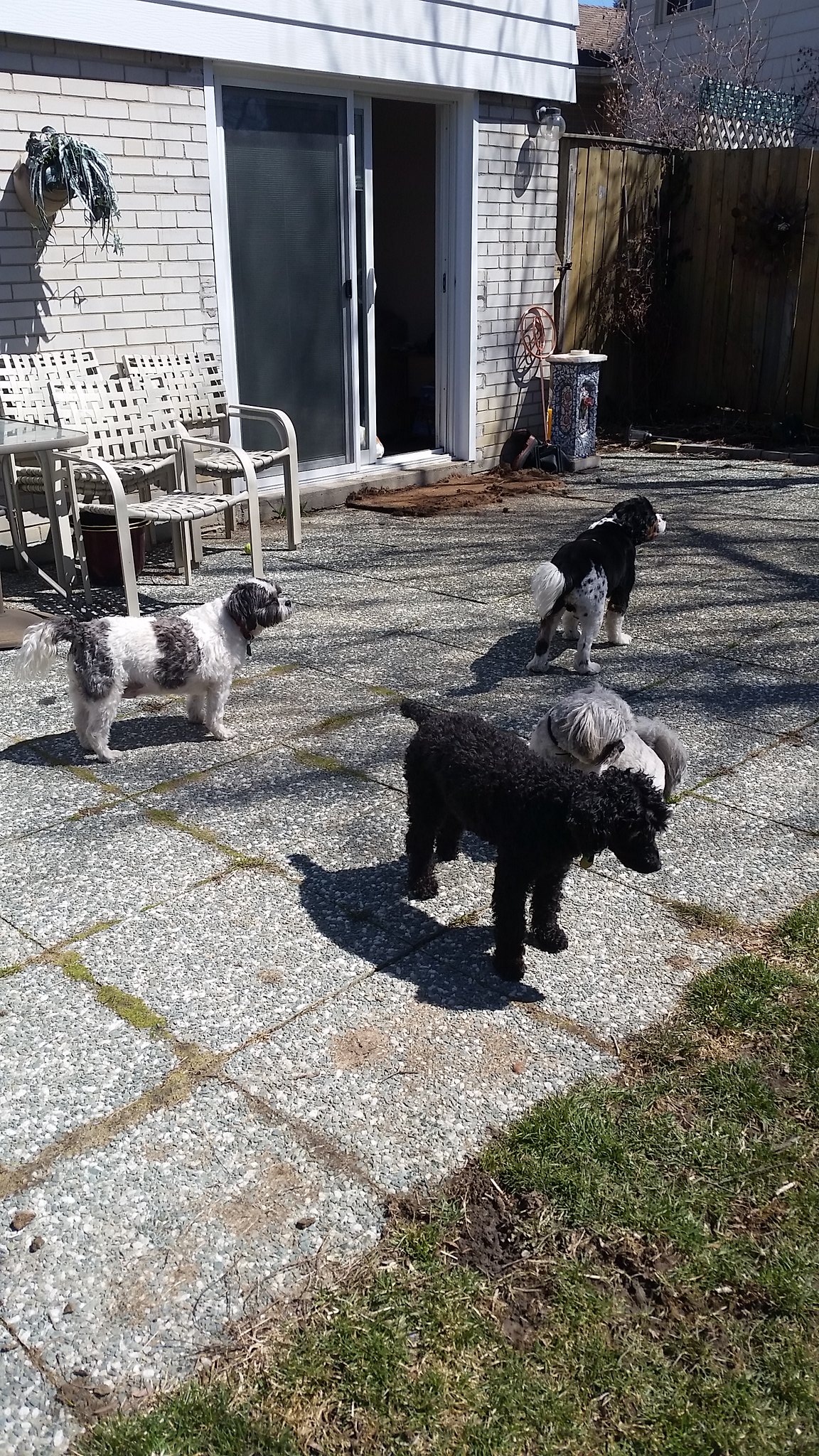The photograph captures a bright, sunny day in a somewhat overcast backyard, featuring a white brick house with an open sliding glass door leading to a spacious patio. The patio, composed of large, pebbly concrete slabs approximately 18 to 24 inches square, shows patches of grass and weeds growing between the cracks. Various pieces of lawn furniture, including worn white deck chairs and a table, are scattered around. There’s also a hanging plant on the building’s exterior, and a brown fence encloses the area. In the lower right-hand corner, a small triangular patch of grass is visible, while the rest of the yard displays soil patches and a scruffy mat near the porch entrance.

In the midst of this scene are four small dogs, some of which are standing close to each other while others are more spaced out. Their colors vary: one is pure black, another mostly white with gray or brown spots, a third is white with black spots, and the fourth gray-colored dog is partially obscured behind the others. Although they’re hard to identify by breed, one appears to be a poodle with a short tail. The dogs seem content, leisurely exploring the patio under the sunlight filtering from the top right of the image.